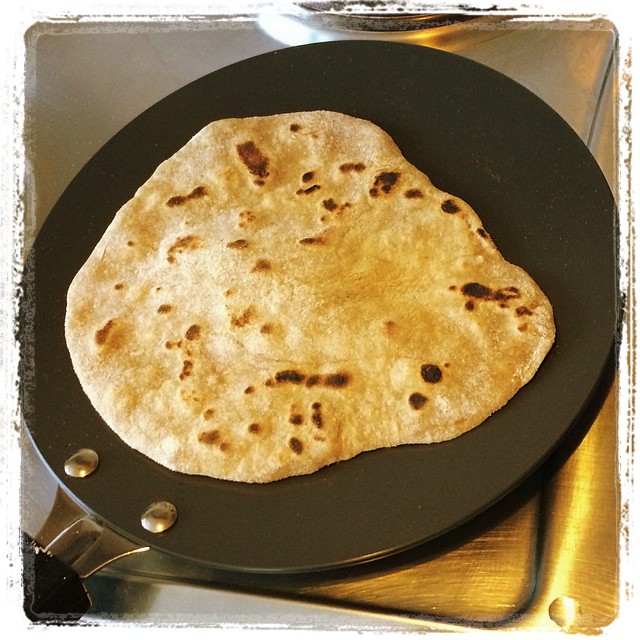This is a full-color photograph likely staged indoors, depicting a culinary scene. At the center of the image is a black frying pan with a partially visible silver handle, transitioning into a black handle at the bottom left corner. The pan holds a handmade tortilla that's been toasted to reveal brown and tan spots, alongside patches of white, indicating different degrees of cooking. This tortilla is circular but slightly irregular in shape. Below and surrounding the pan, the surface is a gray stovetop. The stovetop occupies the entire background, framing the frying pan and the tortilla in a distressed, metallic setting. This image appears to capture the moment of someone cooking on a stove, focusing on the tortilla as the main subject being heated.